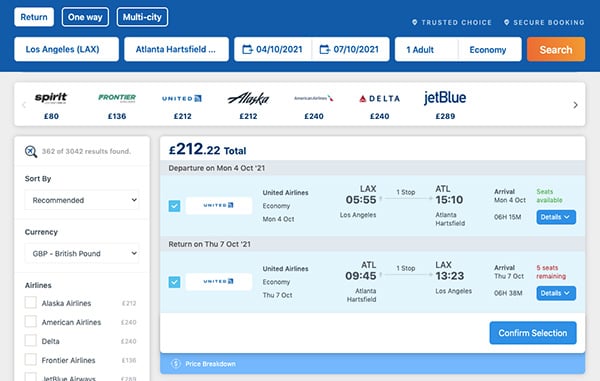This is a detailed screenshot of a flight booking website interface.

In the top left corner, there are three selectable buttons: the first button, indicating a return flight, is white with blue text; the second and third buttons, which represent 'One Way' and 'Multi-City' options respectively, are blue with white text. The background of the main section is a calming blue.

On the right side, there are texts indicating "Trusted Choice" and "Secure Booking." Below this area, there are four input sections: the first displays the departure airport as Los Angeles (LAX), and the second displays the arrival airport as Atlanta Hartsfield (ATL). The next two sections allow users to select travel dates, which have been chosen as April 10th, 2021, for departure and July 10th, 2021, for return. The trip is for one adult in economy class. An orange 'Search' button is prominently displayed below these inputs.

Following this, there is a list of available flights from various airlines, starting with Spirit Airlines at £80, Frontier at £136, United at £212, Alaska Airlines also at £212, American Airlines at £240, Delta at £240, and JetBlue at £289.

On the left side of the interface, there's a section for users to fine-tune their search results. In the center of the page, the selected flight is highlighted, priced at £212.22 in total. The details note that the departure is scheduled for Monday, October 4th, 2021. The outbound flight is with United Airlines, departing from LAX at 5:55 AM, making one stop, and arriving at ATL at 3:10 PM. A dropdown button offers additional details about seat selection.

The return flight is on Thursday, October 7th, 2021, departing ATL at 9:45 AM and arriving back at LAX at 1:23 PM. The interface indicates that only five seats remain available. There is a button to confirm the selection, completing the booking process.